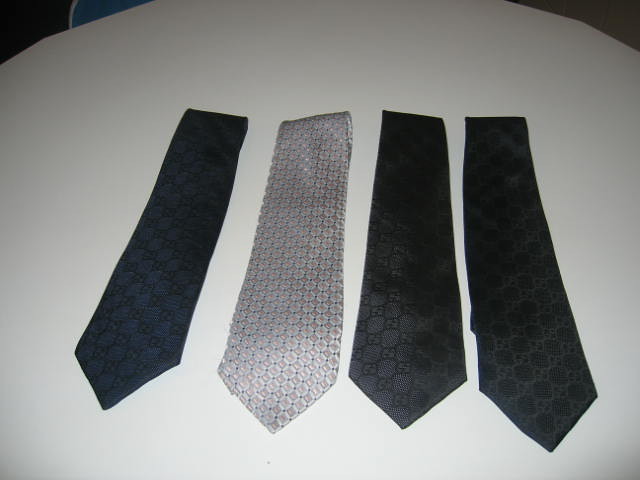The photograph is an amateur close-up shot of four partially folded neckties laid out on a white surface, possibly a table, with a black background framing the upper left and right corners. The image, taken slightly from above with a flash, shows the ties centered but somewhat dark around the edges. The first tie on the left is a navy blue with a honeycomb pattern. Next is a silver tie featuring a light pattern with blue tiny dots. The last two neckties are black, each adorned with subtle, circular patterns. While the photograph is slightly undercropped and dim, it distinctly captures the details and textures of the four neckties.